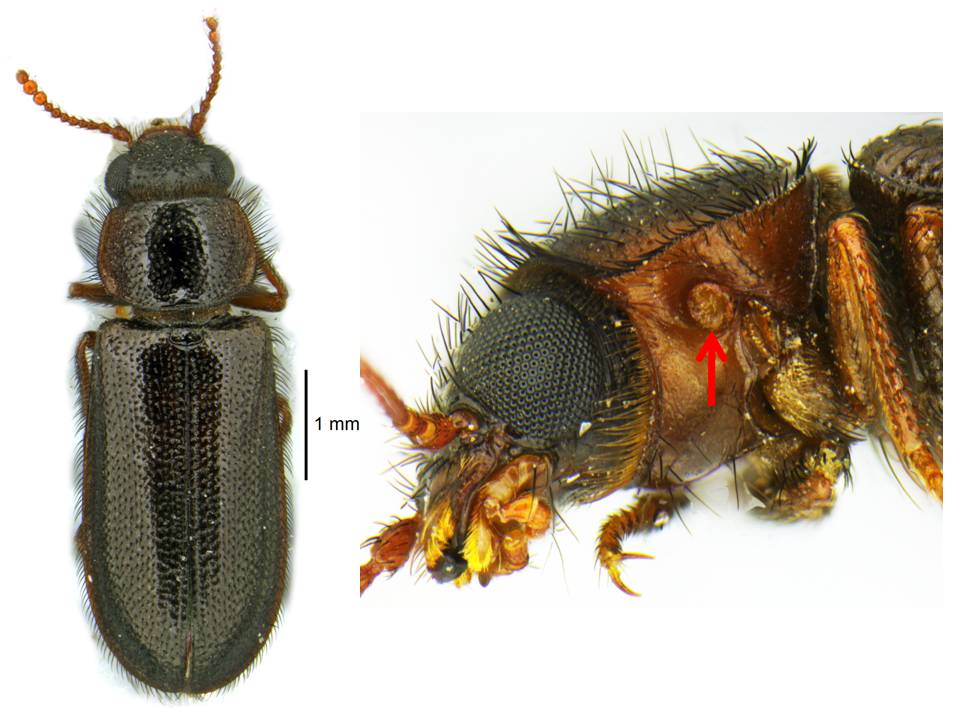The image showcases a small insect, likely a beetle, captured in two distinct views side-by-side for detailed examination. On the left, a top-down perspective reveals the beetle's gray body adorned with orangey antennae and fine, prickly hairs edging its form. There's a one millimeter scale bar indicating the insect's minute size. To the right, a close-up of the insect's face emphasizes its intricate features: brown compound eyes located on the sides of its head, a black snoot, and vivid yellow and orange mouthparts. The head appears more brownish in the close-up than in the top-down view. An arrow points to a specific, albeit unlabeled, part of the insect's face, possibly the eye. The creature has multiple legs with four positioned prominently at the back, and its midsection is notably darker, almost black. Overall, the insect is depicted in scientifically rich detail, combining various angles and close-ups to offer a comprehensive view for study.